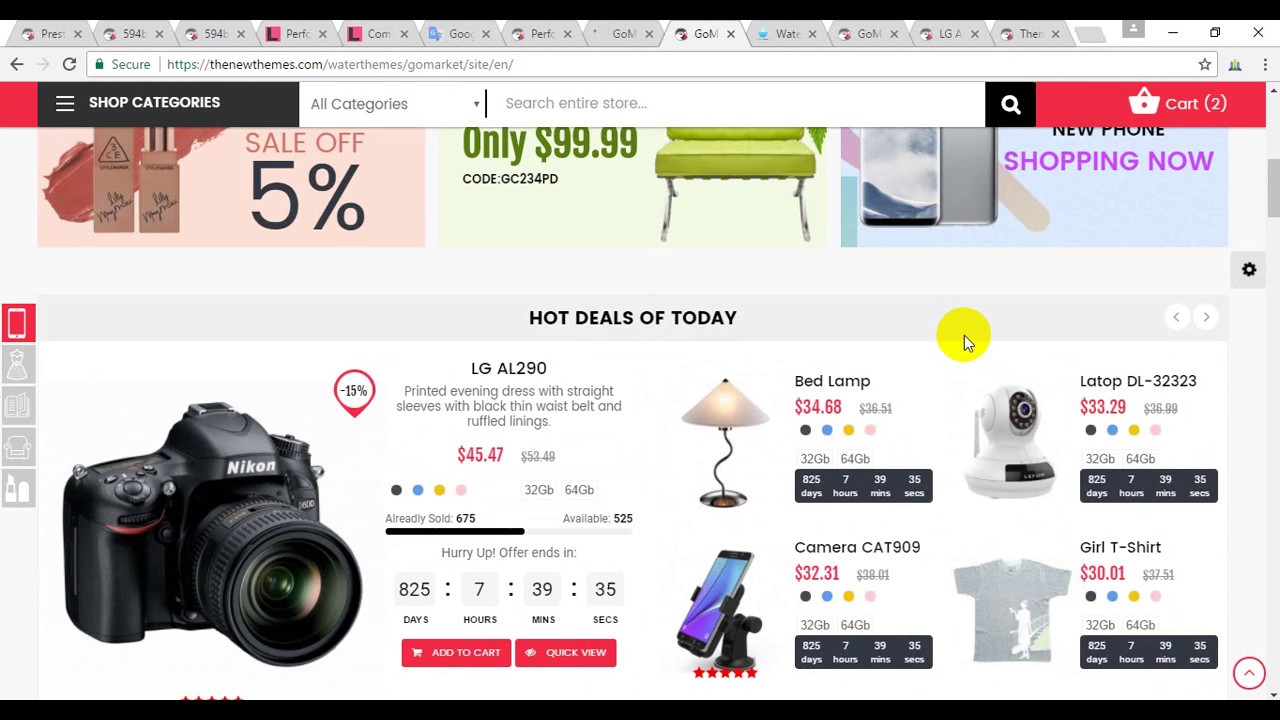This image depicts a detailed screenshot of an e-commerce website. The webpage is framed by a black border at the top and bottom. At the top of the page, 13 different tabs are open, each displayed against a light gray background. Below this, the navigation bar includes a left arrow key in darker print, a faded right arrow key, a refresh symbol, and the text "Secure HTTPS" followed by the web address and a star icon for favoriting the page.

The main section of the website starts with a small red square on the left, followed by a black banner that reads "Shop Categories" in bold text. Below this banner, there is a gray background with darker gray text that says "All Categories." A dropdown menu is indicated underneath. Next to this, there is a search bar with the text "Search Entire Store" next to a black square containing a white magnifying glass icon. To the right, a red banner features a shopping bag icon and the text "Cart (2)" in parentheses.

The body of the website displays several product images on a white background, including a camera, a cell phone, a lamp, a laptop, another camera, and a t-shirt.